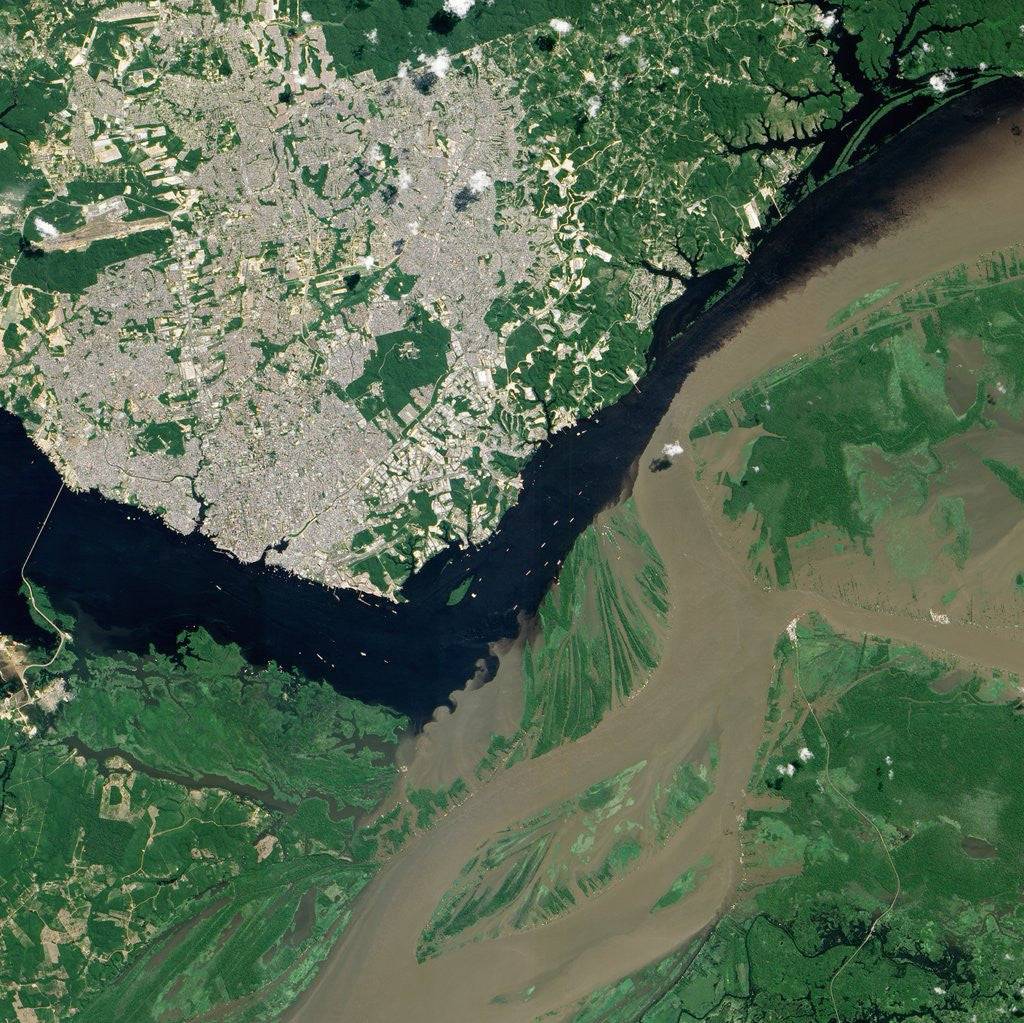An aerial, potentially satellite shot, captures the Earth with remarkable detail, showing a V-shaped river that diagonally traverses from the top right to the bottom left before curving left in the middle. Below this river, the landscape is predominantly green, suggesting a rich natural environment with possible trees and vegetation, along with some brown soil areas. There are sparse white structures that resemble buildings against the greenery. Above the river, extending especially towards the left, lies a cityscape marked by geometric streets and white areas hinting at buildings, interspersed with patches of greenery. This urban area covers approximately two-thirds of the upper left side. In contrast, the right side of the image predominantly features natural landscapes, with possible signs of striations indicating past flooding or mudslides in the lower part.